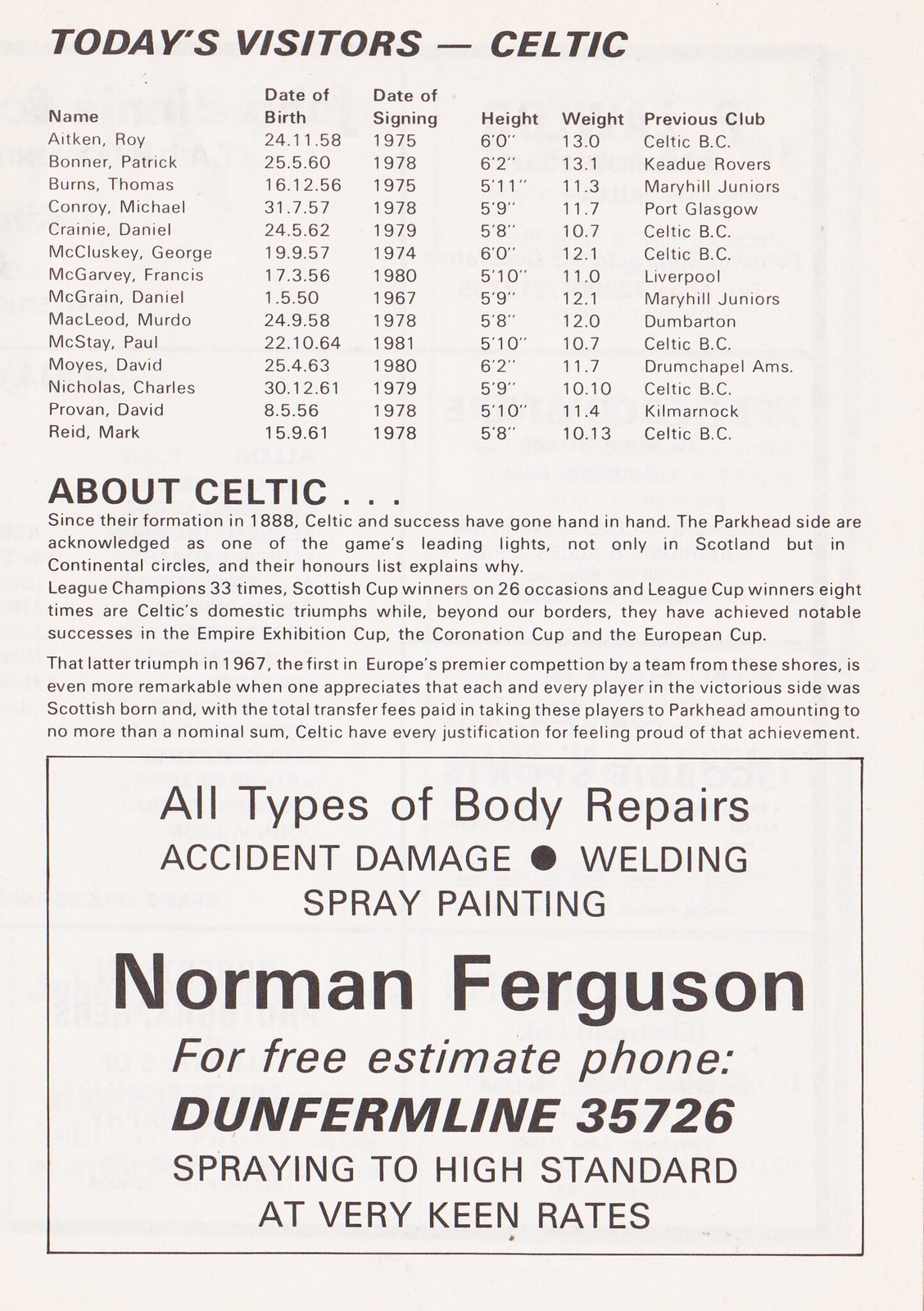This image depicts a page from an aged football (soccer) program, which is slightly discolored from its original white to an off-white hue. The page is divided into three distinct sections. At the top, in bold capital letters, it reads "Today's Visitors, Celtic". This section features a comprehensive roster of Celtic players listed alphabetically, including detailed information such as their date of birth, date of signing (mostly from the 1970s and early 1980s), height, weight, and previous clubs.

The middle section is titled "About Celtic" and delves into a brief history of the team, highlighting the club's formation in 1888 and emphasizing its longstanding success.

At the bottom of the page is an advertisement for auto body repair services. It offers a range of services including accident damage repair, welding, and spray painting. The ad features the name Norman Ferguson, and provides a contact number—Dunfermline 35726—along with a promise of high-standard service at competitive rates.